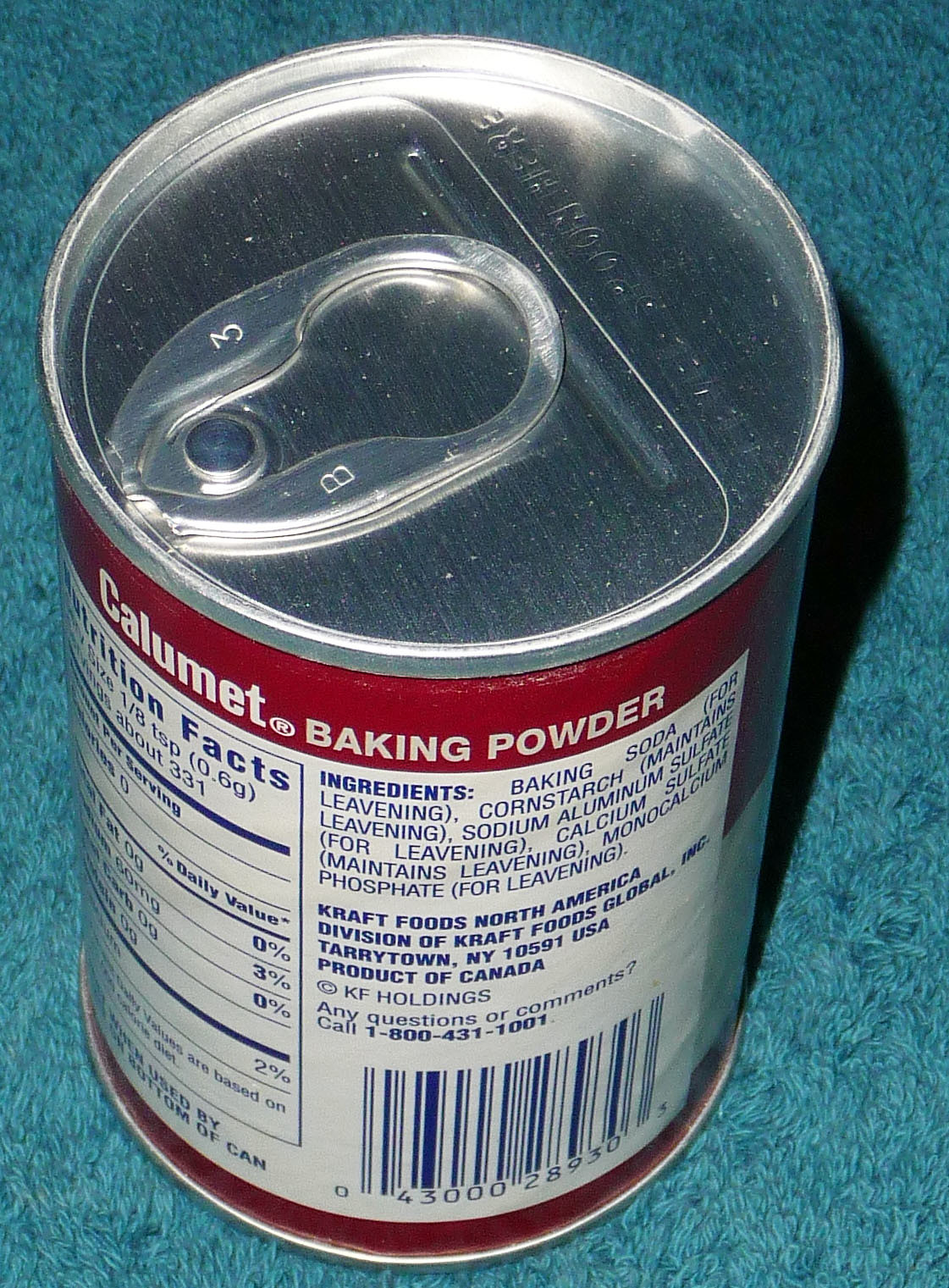The image depicts an aluminum can with a pop-tab top, prominently labeled as "Calumet Baking Powder." The brand name "Calumet," spelled C-A-L-U-M-E-T, is clearly visible on the can, which features a red and white label. The ingredients listed on the can are as follows: baking soda (for leavening), cornstarch (maintains leavening), sodium aluminum sulfate (for leavening), calcium sulfate (maintains leavening), and monocalcium phosphate (for leavening). The label also indicates that the product is manufactured by Kraft Foods, North America, a division of Kraft Foods Global Inc., and provides a 1-800 contact number. The can is placed on blue carpeting.